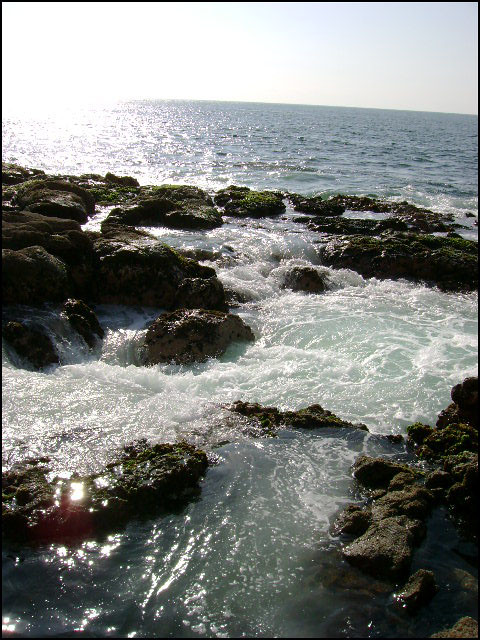This photograph captures a serene coastal scene where the open ocean meets a rugged, rocky shoreline. The top of the image showcases a vivid blue sky, interspersed with patches of bright white light reflecting off the ocean's surface, particularly towards the left where the sun is visible. Below the sky, the expansive, blue ocean stretches out until it meets an area filled with black and gray rocks, roughly 60% down the picture. Among these rocks, the water becomes frothy and white, swirling and bubbling as it flows through the rocky terrain. The left side of this rocky region is densely packed with rocks, while the right side has fewer rocks and more frothy, turbulent water. Towards the bottom of the image, the water calms, becoming still and clear, reflecting the sunlight glinting off the damp rocks and revealing patches of algae. The overall image has a slight clockwise tilt, adding a dynamic feel to the tranquil beach scene.